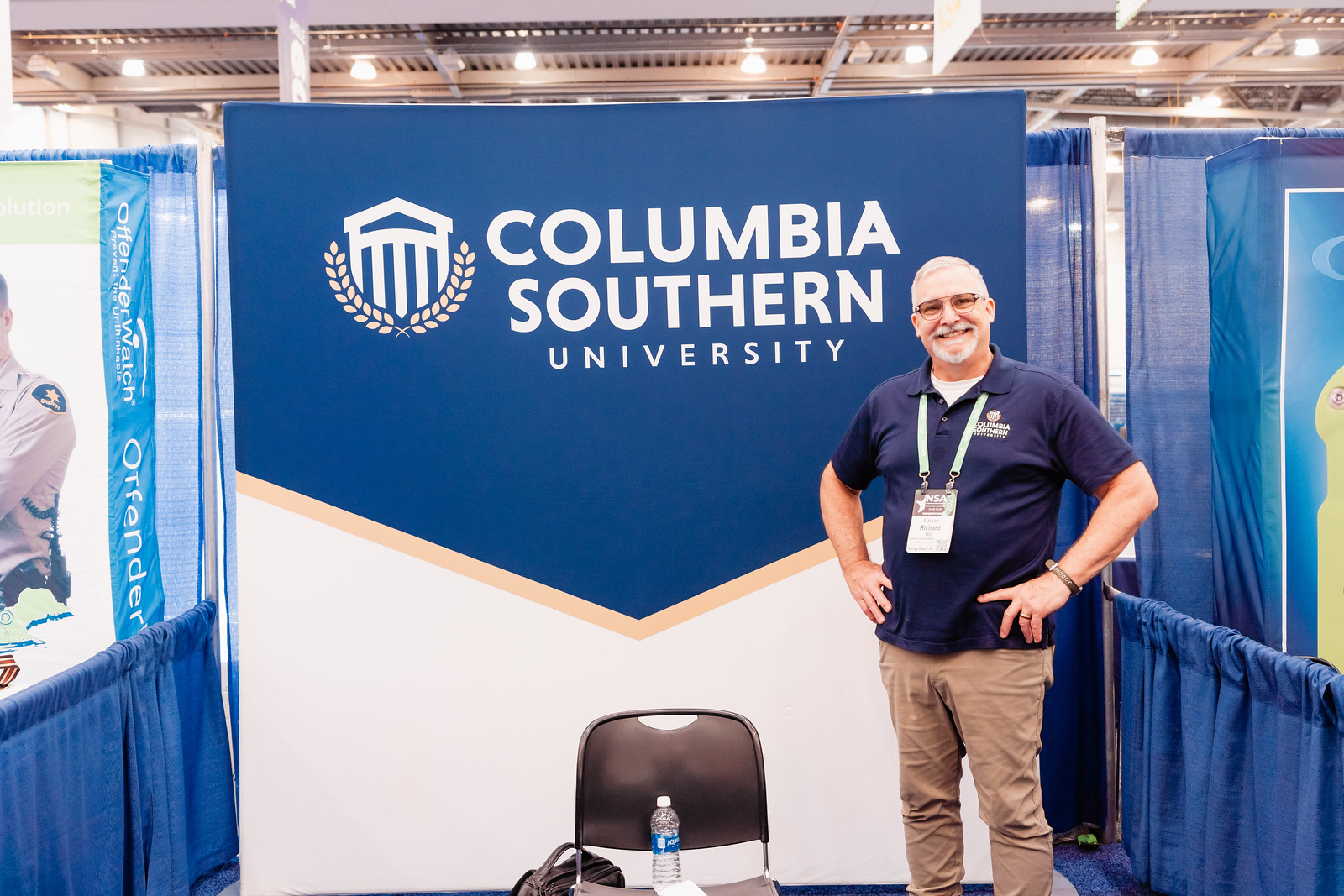This detailed indoor photograph captures a smiling, older Caucasian man with white hair, a white beard, and mustache. He is wearing dark-rimmed glasses, a navy blue short-sleeved polo shirt, a lanyard with an ID around his neck, and long brown pants. He is standing slightly to the right of the center of the image with his hands on his hips. 

In the middle of the photo, there is a gray metallic folding chair with a water bottle placed on top of it. Behind the man, there is a large banner, predominantly navy blue on the top half and white on the bottom, separated by a strip of yellow or gold. The banner displays the text "Columbia Southern University" in white letters, along with the university's logo of a sloped roof column building with gold laurel leaves beneath it.

The indoor setting is illuminated by metallic ceiling lights and features blue cloth curtains creating separate display areas on the left and right sides. Another banner depicting a police officer is visible in the left-side section, indicating this is likely an event space with various sectional displays.